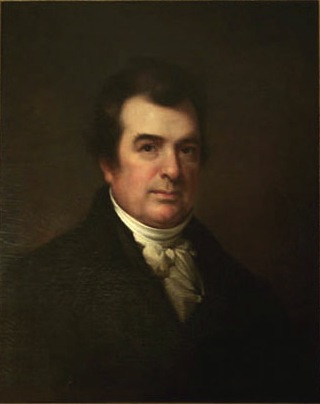The image portrays a middle-aged man, likely in his 50s, with very fair skin and a slightly receding hairline. His dark brown hair is short but somewhat poofy, enough to cover his ears and stick up slightly. He has dark brown, heavy eyebrows and a neutral expression on his face, with his mouth closed. There's a hint of redness on his cheeks and just under his eyes. He appears to have a bit of heaviness around his chin, possibly indicating a slight double chin.

He is dressed in period attire suggestive of the 1800s. He wears a heavy brown or black jacket with visible lapels, over a tightly wrapped white shirt that extends firmly around his neck and down his chest. The shirt features a white bow tie, made of the same material, though it blends in and is slightly difficult to discern. Behind him, the background is a gradient of dark colors, primarily brown or light black, with slight hints of green. The portrait, painted in a traditional style, captures the stoic and serious demeanor of the man, emphasizing the fashion and artistic techniques of the era.